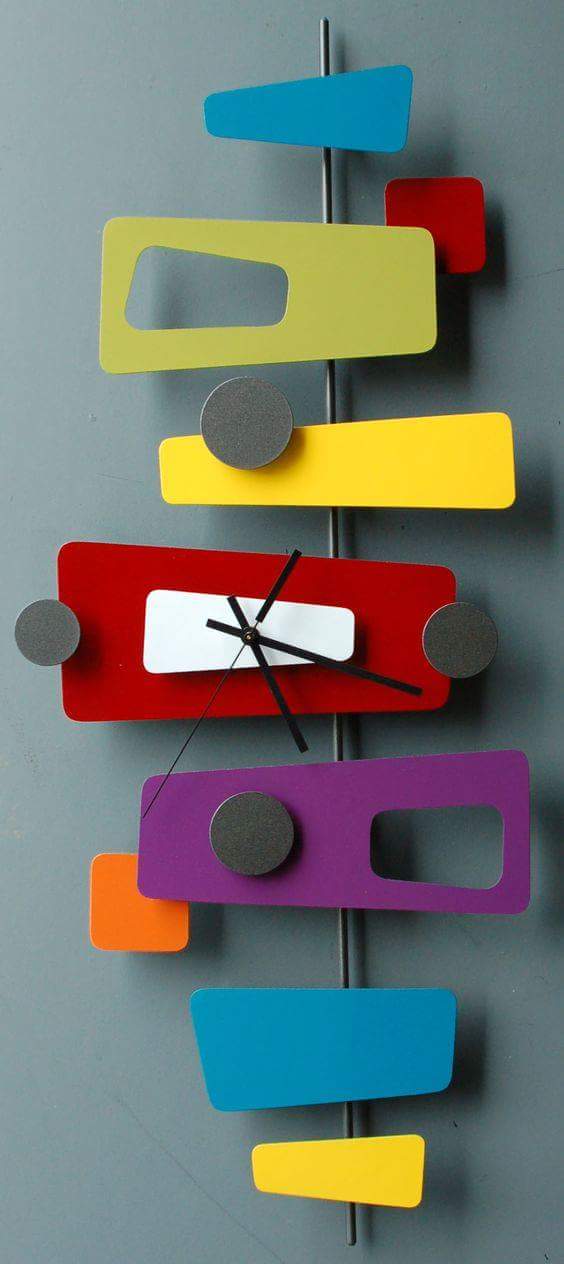The image portrays a unique xylophone-inspired clock set against a gray background. The central element of the composition is a metallic stick that thickens towards the top, serving as the primary support structure. Arranged horizontally across the stick are five or six rectangular pieces, reminiscent of xylophone bars, suggesting they are made out of plastic. Positioned at the center of this configuration is a clock face embedded in one of these rectangular bars. The clock, crafted with precision, features black hour, minute, and second hands. The hands are all pointing to indicate the time as approximately 5:17. This inventive design seamlessly blends elements of music and timekeeping, creating a visually striking and functional art piece.